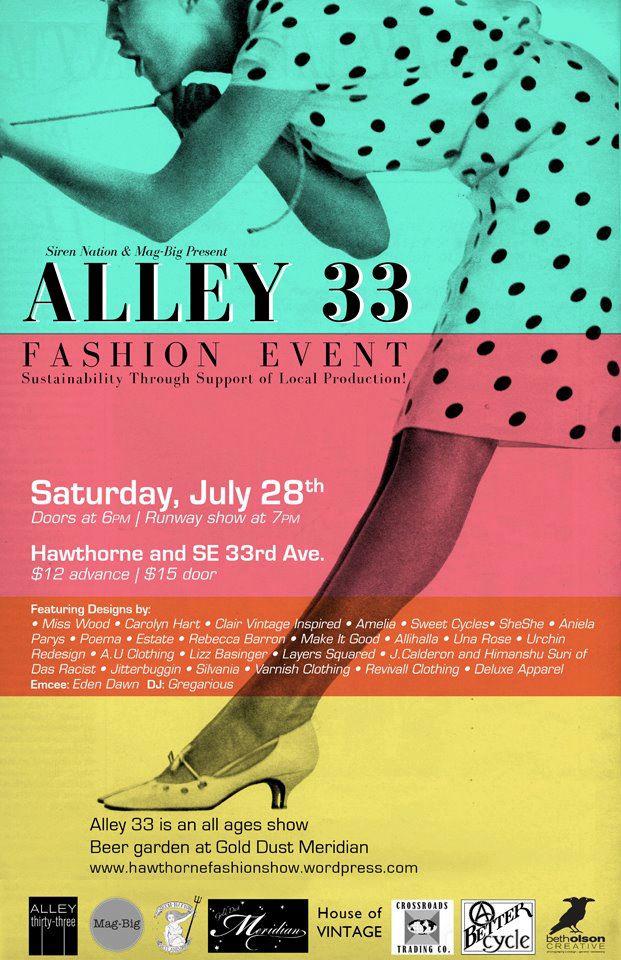This detailed advertisement features an event announcement for the "Alley 33 Fashion Event," focusing on sustainability through supporting local production. The advertisement sports a vibrant color scheme with mint green, peach, and yellow blocks going down from top to bottom. A woman in the vintage style of the 1960s is depicted, bent over and pulling a string while dressed in a classic polka dot dress and white small heeled shoes. Overlaid on the image are the event details: "Siren Nation and MAG Big present Alley 33 Fashion Event, sustainability through support of local production." The event date is listed as "Saturday, July 28th, doors at 6 p.m., runway show at 7 p.m.," at the location "Hawthorne and SE 33rd Avenue." 

Ticket prices are specified as "$12 advance, $15 door." The advertisement features a long list of designers including Miss Wood, Carolyn Hart, Claire Vintage Inspired, Amelia Sweet Cycles, She She, Anila Perry's Poma Estate, Rebecca Barron, Make It Good, Ali Hala, Una Rose, Urchin Redesign, AU Clothing, Liz Basinger, Layers Squared, Jay Calderon, and Himanshu Suri of Das Racist. Additional contributors such as Jitterbug in Sylvania, Varnish Clothing, Revival Clothing, Deluxe Apparel, MC Eden Dawn, and DJ Gregarious are also highlighted. It is noted that the "Alley 33 is an all ages show," with a "Beer Garden at Gold Dust Meridian."

At the bottom of the advertisement, a row of sponsors is displayed, including A Better Cycle, House of Vintage, Alley, and Magbig, along with various icons representing event sponsors. The website for more information is provided as "www.hawthornefashionshow.wordpress.com."